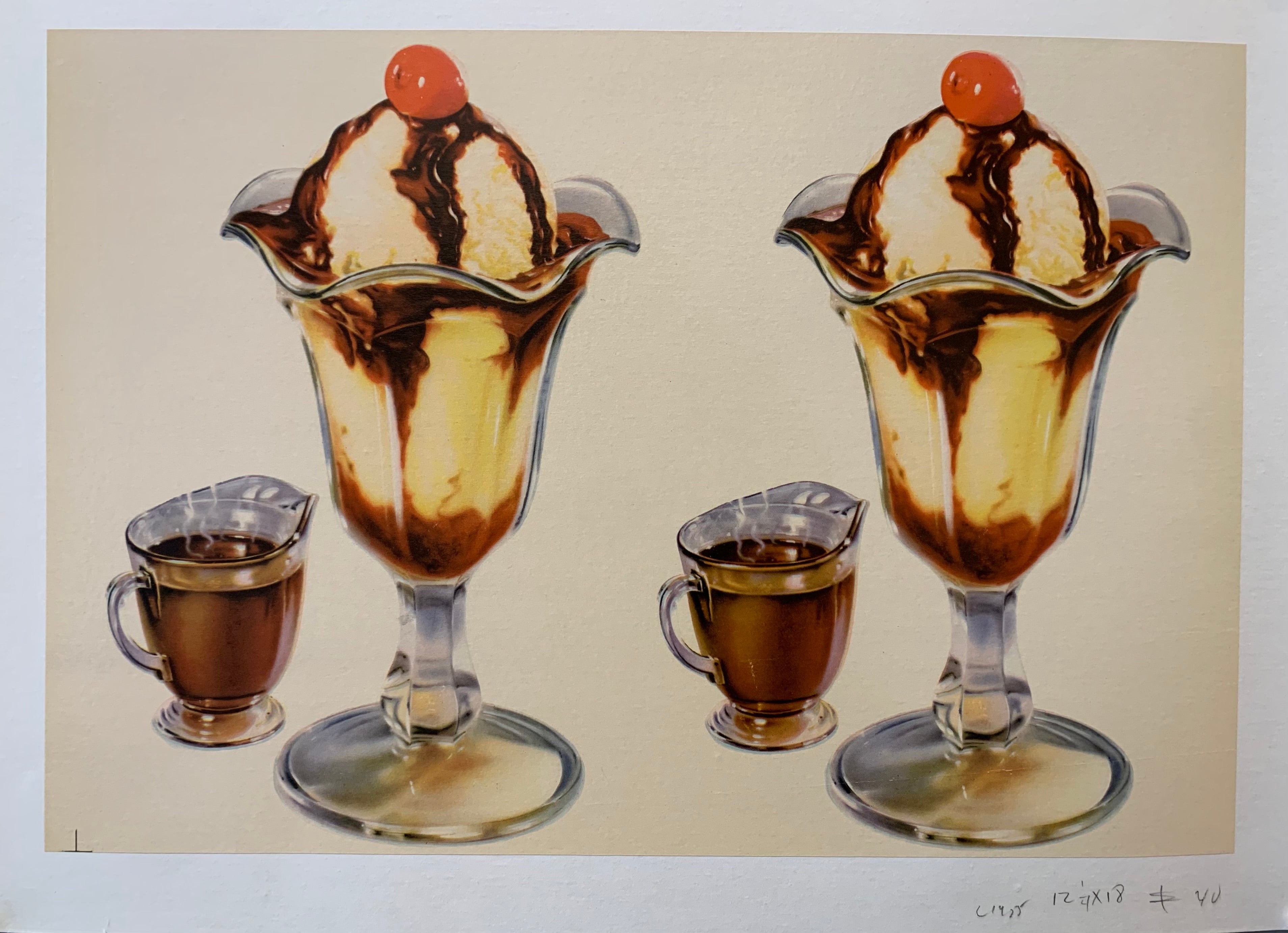The image depicts a detailed and elegant arrangement of two identical cherry sundaes, each nestled in ornate glass goblets with wide bases. Each sundae showcases layers of rich vanilla ice cream, artfully streaked with cascading lines of chocolate syrup. Crowned with a glossy red cherry, these sundaes exude a classic appeal. To the left of each goblet, there are small glass pitchers brimming with chocolate syrup, inviting the viewer to indulge further. The backdrop is a soft, cream-colored hue, enhancing the visual charm of the scene. The image, possibly serving as an advertisement, features some text and numerical figures along the bottom, which may include the artist's name and dimensions of the artwork. The entire composition rests gracefully on a countertop, creating an inviting and nostalgic ambiance.